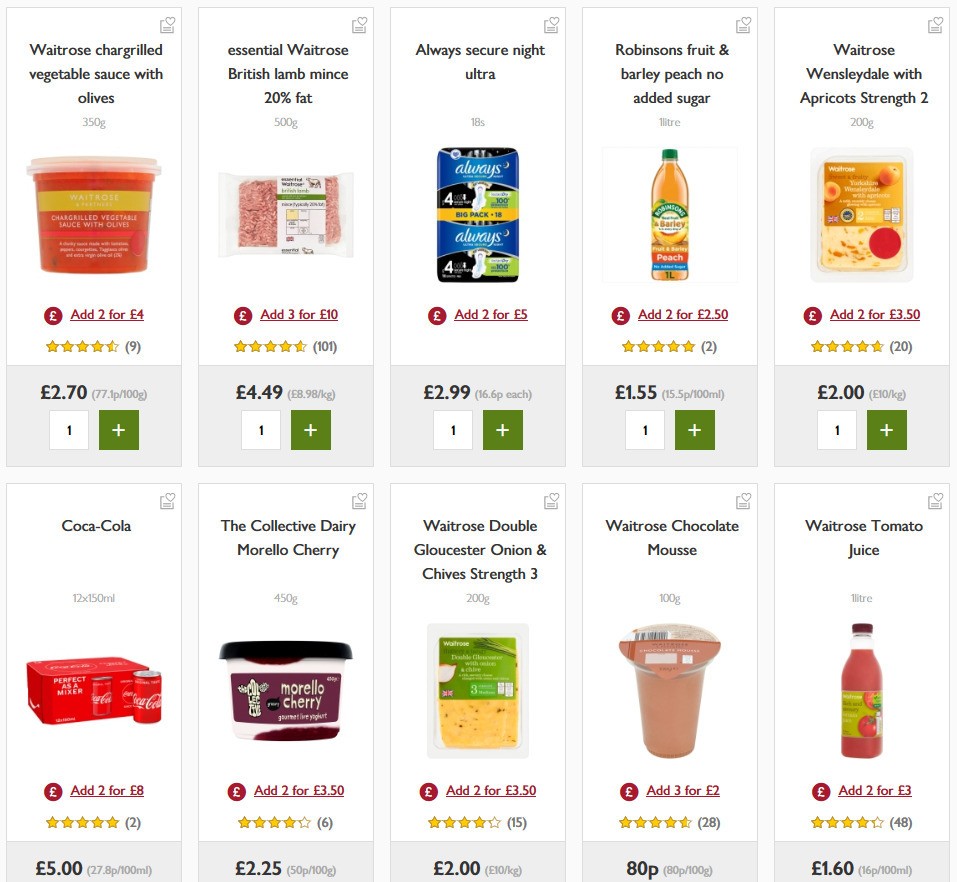The image displays a section of an e-commerce grocery store website, featuring a variety of products available for purchase. The website header and the store's name are not visible in the frame. Each product listing includes a thumbnail image, the product name, and a star rating based on customer reviews. Below the star ratings, there is an interactive gray box indicating the current quantity selected, alongside a white box where customers can specify the desired amount. Additionally, a plus sign is provided to easily increment the number of items to be added to the cart.